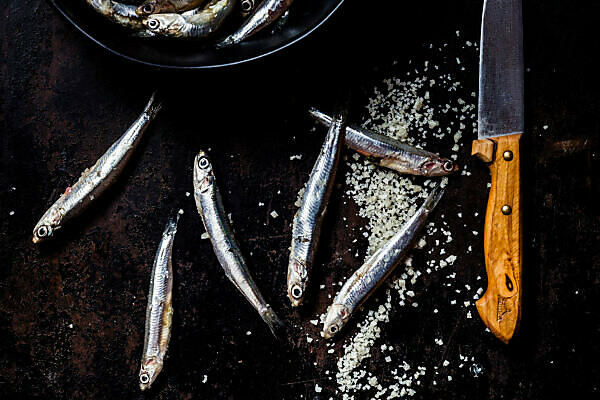A rectangular photograph taken from an overhead angle captures a scene centered on a mottled black and brown tabletop surface. In the middle of the image, there are six slender, small fish, exhibiting a brown-silver sheen, likely sardines or smelts. Their distinctive eyes feature a round black circle surrounded by a white ring, with a black dot at the center. The fish lie on a textured layer of white, gravel-like material. To the right side of the image, a short knife with a brown wooden handle is visible, secured by two golden screws. This knife is positioned close to two of the fishes, which rest on the white gravel. At the top of the image, the partial edge of a black plate or saucepan intrudes into the frame, containing more of these fish. The lighting, though not optimal, adequately illuminates the scene. Additionally, a semi-transparent gray watermark featuring the letter "M" within a circle is noticeable at the bottom center of the photograph.